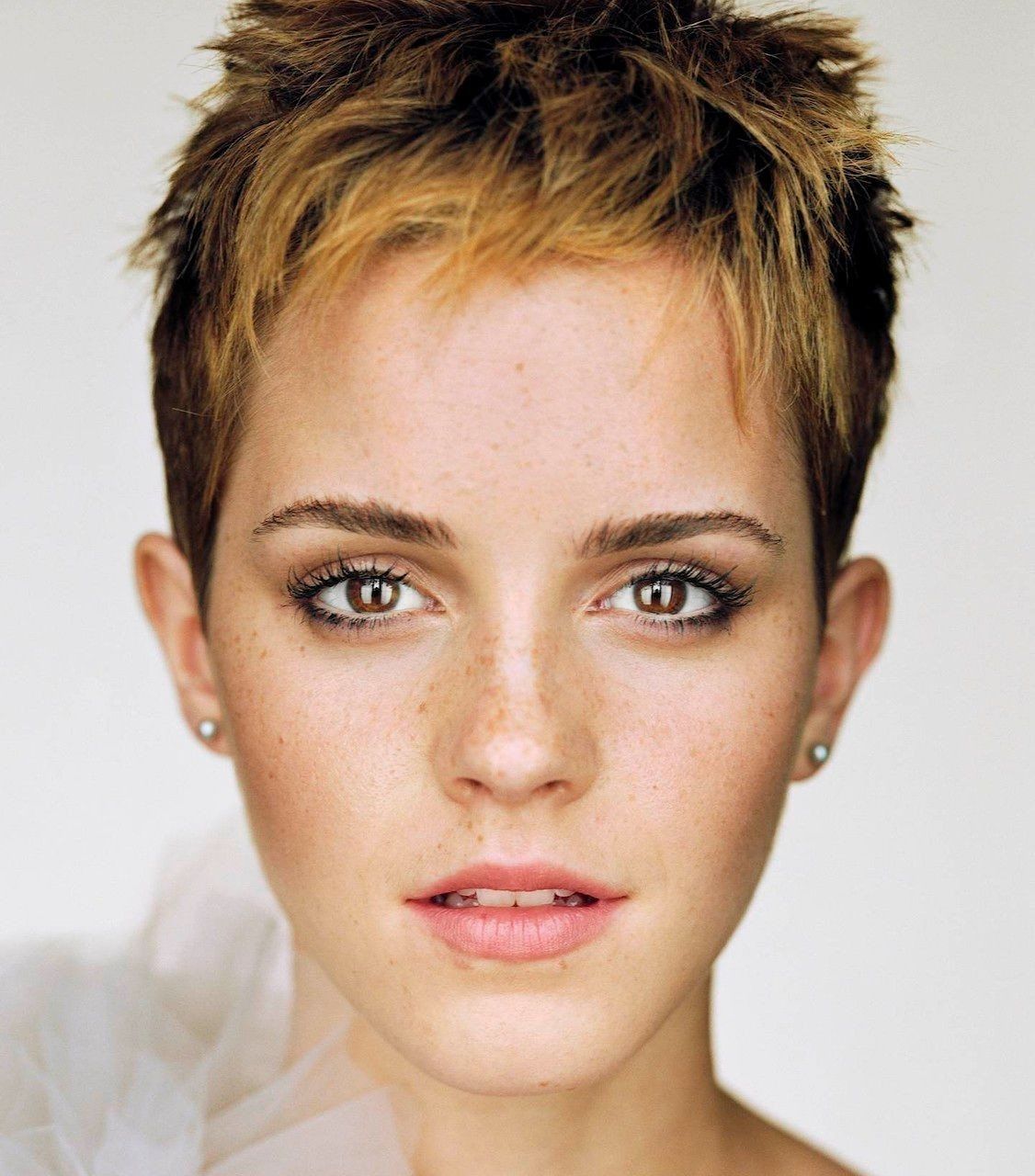This is a very detailed headshot of a young woman, likely in her 20s, with an impeccably made-up face. She is looking straight at the camera, giving the impression of a professional, close-up modeling shot. Her short, pixie-cut hair has a striking appearance with dark roots and lighter, blondish-red tips. Her skin carries an olive tone yet appears fair, adorned with slight freckles across her nose, cheeks, and temples, adding to her delicate beauty. 

The woman's eyes are a rich chocolate brown, accentuated with mascara, and her eyebrows are perfectly manicured. She wears light pink lipstick that complements her natural look. Small steel or silver stud earrings glint subtly at her ears. The background is white, creating a clean and distraction-free focus on her face. 

She is dressed in a delicate, possibly chiffon or white opaque lace garment, visible at the top of her shoulder near her chin. The styling, including her muted makeup and the clear visibility of her freckles, enhances her youthful and fresh appearance.